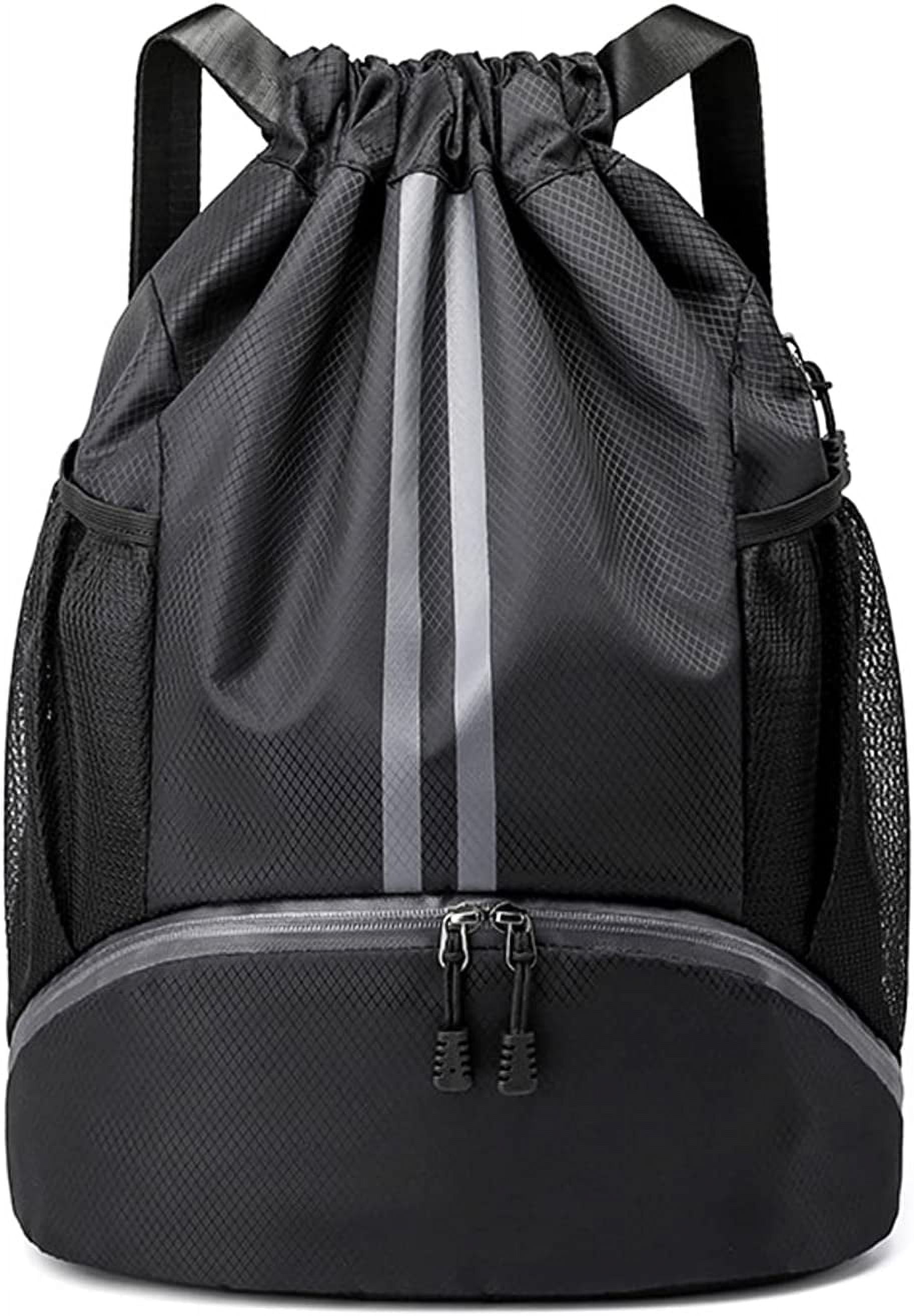This image, a portrait-oriented color photograph, showcases a high-end, black backpack made from a sleek, mesh-like material, giving it a high-tech, almost carbon composite appearance. The backpack is positioned vertically, seemingly floating in a featureless white void, indicative of commercial product photography intended for online shops or catalogs to focus attention solely on the product. The bag features a cinched, drawstring top that is currently closed, flanked by two shiny black shoulder straps. Dominating the design are two prominent silver stripes running vertically from the top to the front pocket. The front is equipped with a silver zipper with black tags attached to the zipper pulls, adding a touch of contrast. On each side of the backpack are mesh pockets, banded at the top with a stretchy material, providing additional storage options. The overall style emphasizes realism and detail, highlighting the backpack's functional and luxurious design.